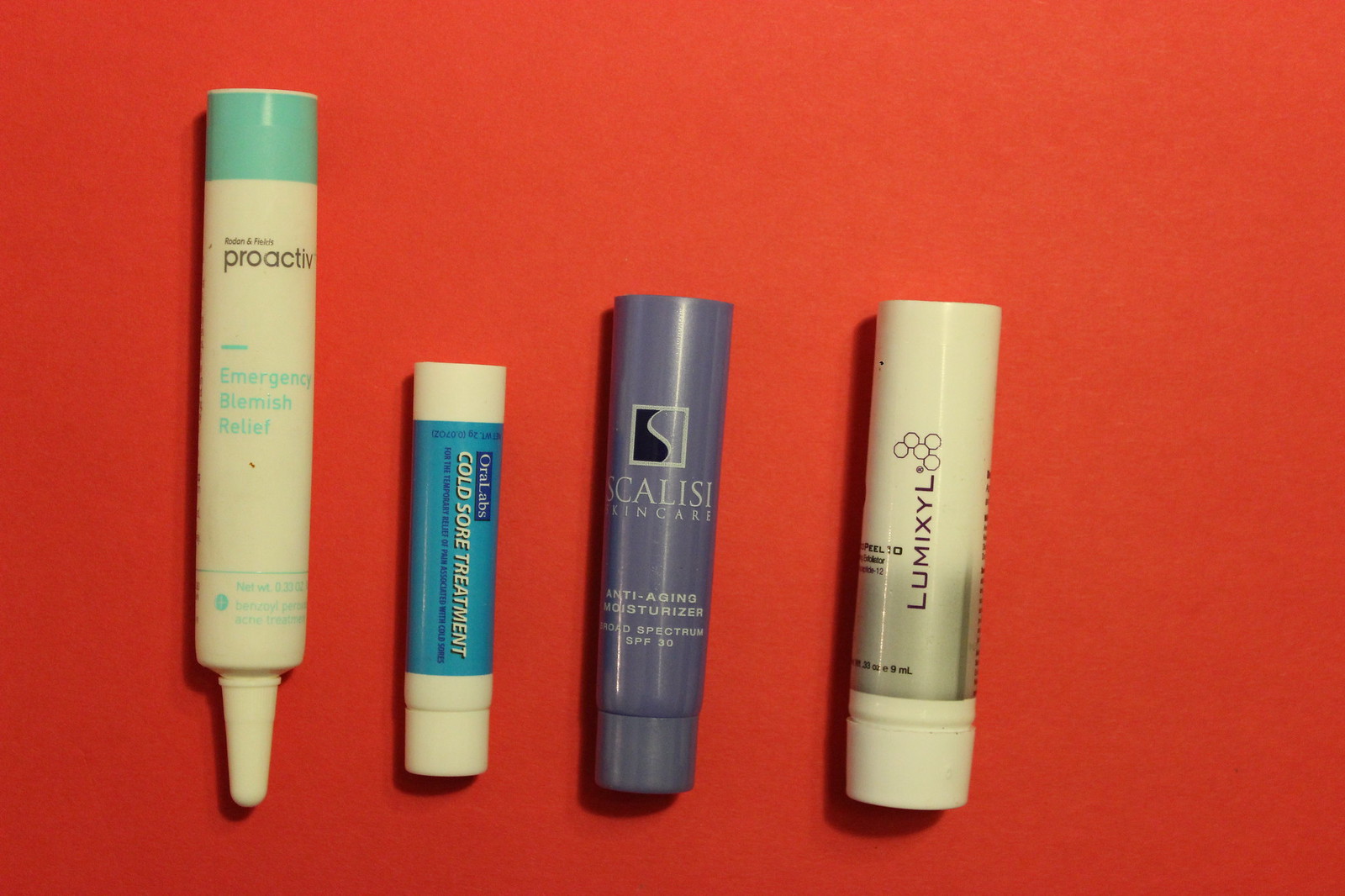This indoor photograph showcases a selection of skincare products arranged against a striking red background. On the far left, a white tube with a teal band at the top bears the brand name "Proactiv" in black letters, along with the product name "Emergency Blemish Relief" in teal letters. Adjacent to it, there is a chapstick-like product in a white tube, featuring a blue label that reads "Cold Sore Treatment" in white letters, capped as a typical chapstick would be. The next item in the lineup is a blue tube labeled with the brand "Gleasy Skin Care" in white letters, advertising its "Anti-Aging Moisturizer." The final product is a sophisticated tube labeled "Lumixil," with the name displayed in bold red letters against a white label that transitions into a gray hue towards the bottom, with the base of the tube being completely gray. The branding "Lumixil" appears in a gradient from black to reddish letters, enhancing its visual appeal.